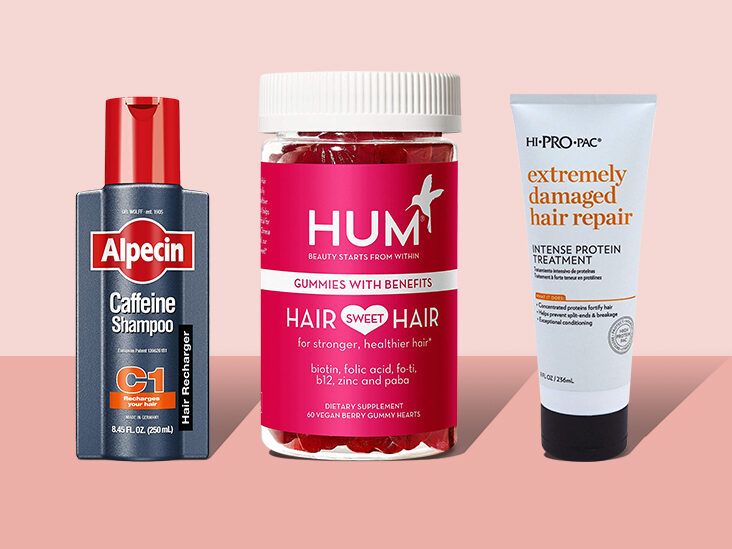The image is an advertisement showcasing three distinct hair care products arranged on a darker pink table against a pale pink wall. On the left is a blue bottle with a red pump top labeled "ALPECIN" in white font on a red background, and "Caffeine Shampoo" below it. It also displays "C1" in orange and "8.45 fl oz (250 ml)" along with "Hair Recharger" vertically. The middle product is a bottle with a white cap and a dark rose label for the brand "HUM." It prominently features a hummingbird outline and the tagline "Gummies with Benefits." The product, named "Hair Sweet Hair," is advertised for stronger, healthier hair with ingredients including biotin, folic acid, B12, zinc, and folate, and contains 60 vegan berry gummy hearts. On the right is a white tube labeled "Hy-Pro-Pak" in orange font, indicating it’s an "Extremely Damaged Hair Repair" cream with "Intense Protein Treatment" written beneath in black font.